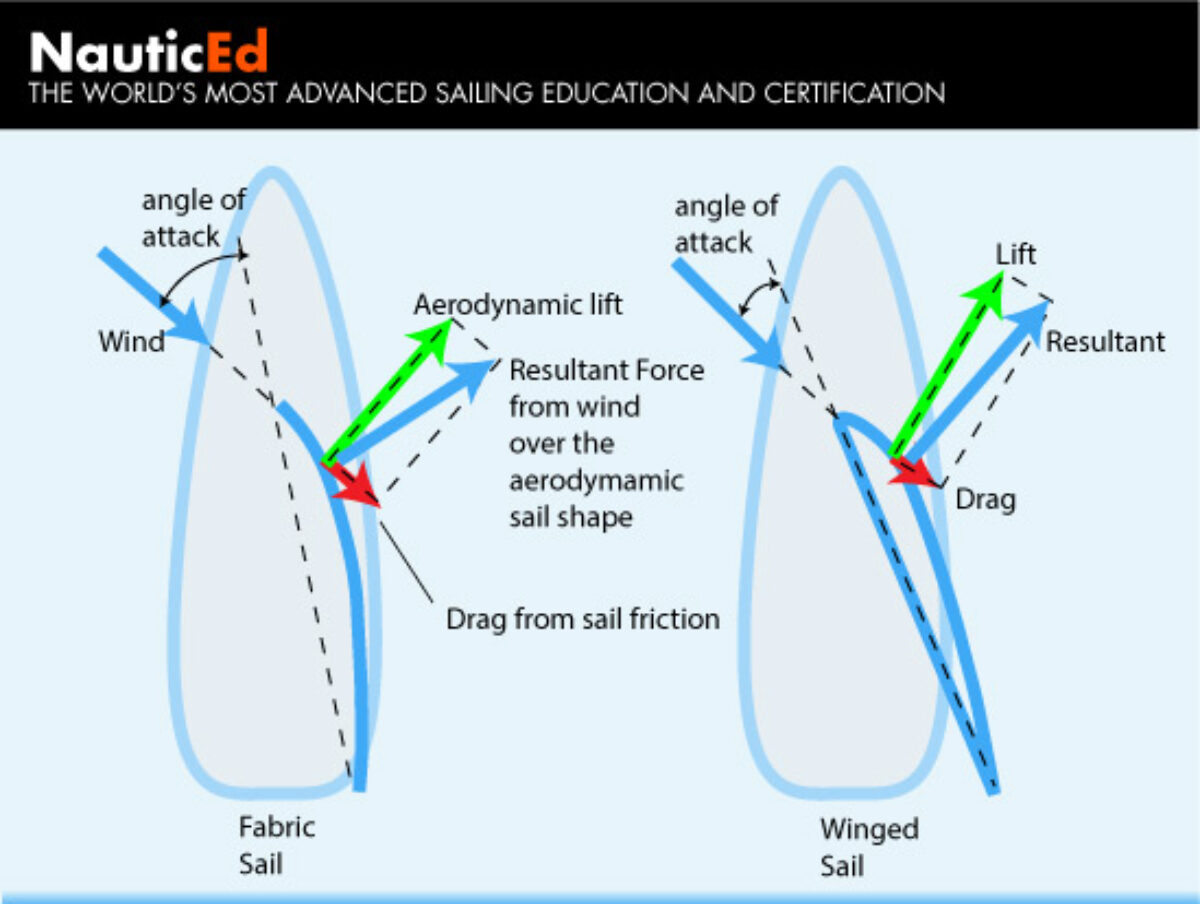The image is a detailed scientific diagram resembling a page from a slideshow or book, illustrating concepts in advanced sailing education. At the top, a black band features white and orange lettering, stating "Nautic Ed" as the world's most advanced sailing education and certification platform. Below this, the diagram itself is split into two sections, each with a light blue oval shape. Both shapes are marked with colored arrows: blue, green, and red. In the center of each oval, text explains aerodynamic principles such as "resultant force from wind over the aerodynamic sail shape" and "drag from sail friction." The left oval is labeled "fabric sail" and the right oval is labeled "winged sail." Additional labels include terms like "angle of attack in wind," "aerodynamic lift," and "resultant force." Both ovals depict the interactions of aerodynamic lift and drag with the sail type.